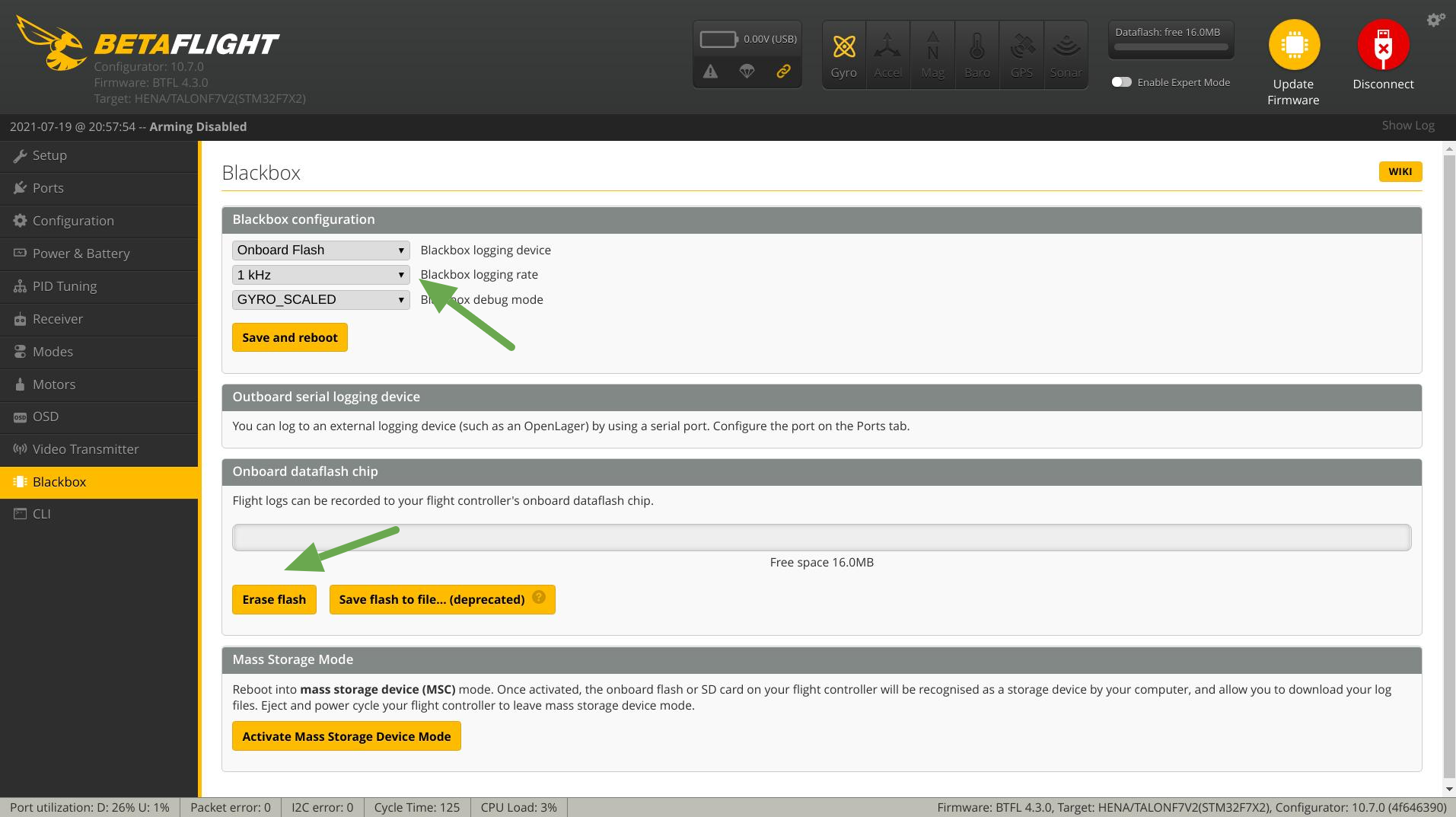This is a screenshot of the Betaflight website interface. The company name is prominently displayed with "Beta" in orange and "flight" in white, accompanied by an orange eagle logo with its wings raised. On the right side, there is a red circle labeled "Disconnect" and a yellow circle labeled "Connect." The top section features various icons within boxes for navigation.

Running vertically along the left side of the interface, there are multiple menu items listed in white text, though they are too small to be clearly legible. Below this, an orange box labeled "Blackbox" is visible. In the central area of the website, the same label "Blackbox" reappears, surrounded by several settings and options.

One section under the "Blackbox" heading is titled "Configuration" and includes a gray arrow pointing toward the middle, where it displays "1 MHz" or "1 Hz." Options such as "Save" and "Reboot" are available here. Further down, there is a reference to an "Outboard Serial Logging Device" with a descriptive write-up.

The next section mentions an "Onboard Data Flash Chip" featuring a green arrow pointing downwards to options like "Erase Flash" and "Save Flash to File," followed by a note that it is "Deprecated." At the bottom of the interface, there is a section titled "Mass Storage Mode" with an orange box prompting users to "Activate Mass Storage Device Mode," along with some additional text in gray.